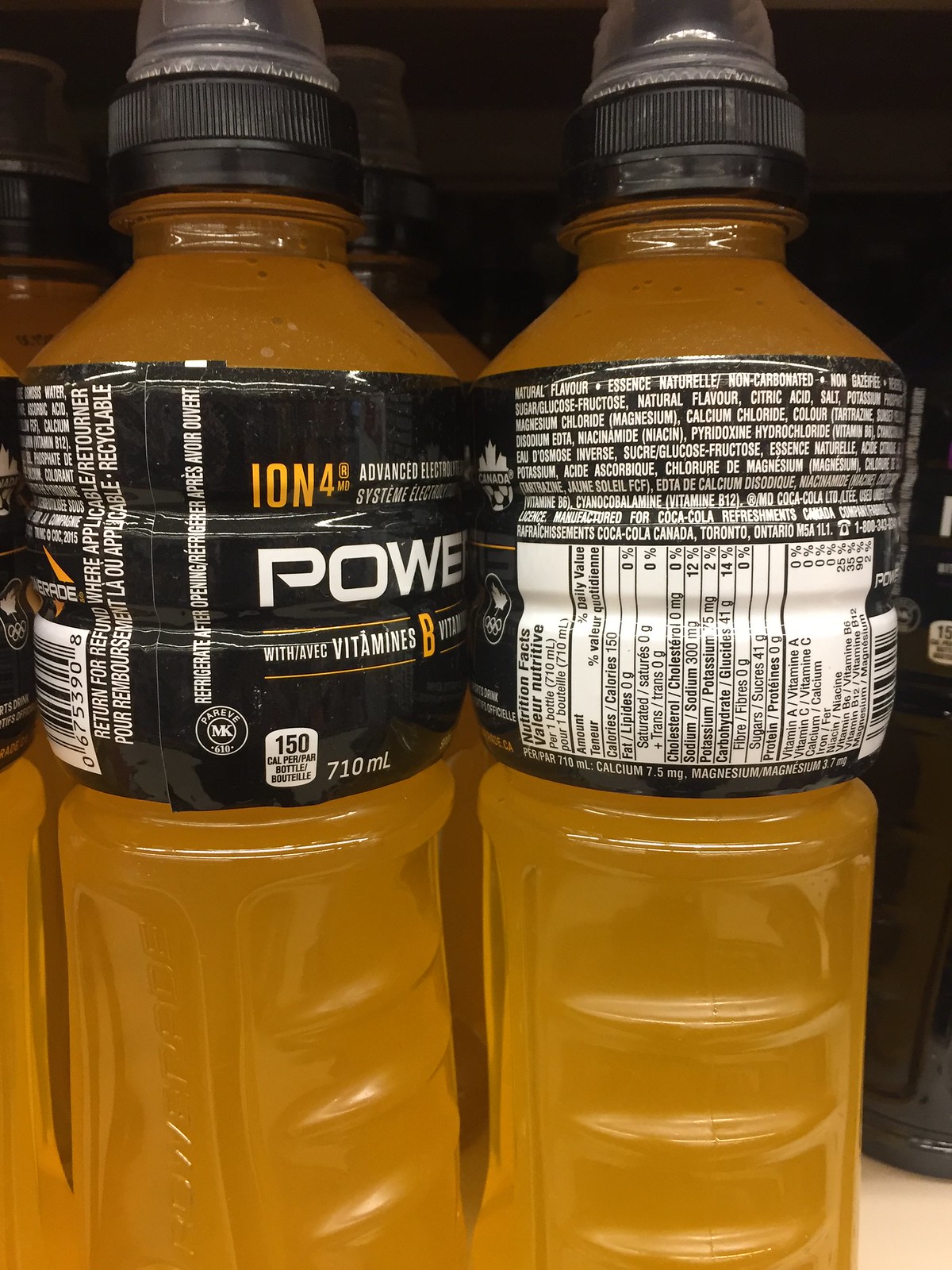The image captures an assortment of Powerade bottles lined up, with the focus on two prominent ones in the foreground. The left bottle is uniquely positioned, showing a partial view of both its front and back. The front displays the text "ION4 Advanced Electro," but the words fade away as the bottle curves. You can also see part of the word "POWER" prominently. Below that, the label mentions "with AVEC Vitamins B," followed by "150, 710 milliliters." The glossy black label creates a subtle reflection, adding a touch of glossiness to the scene.

The right bottle, on the other hand, is angled to prominently display its nutritional information and ingredients list, written in both English and another language. Behind these two central bottles, more Powerade bottles can be seen to the left, adding depth and context to the setting. The overall composition and details highlight the branding and packaging elements of the Powerade bottles.